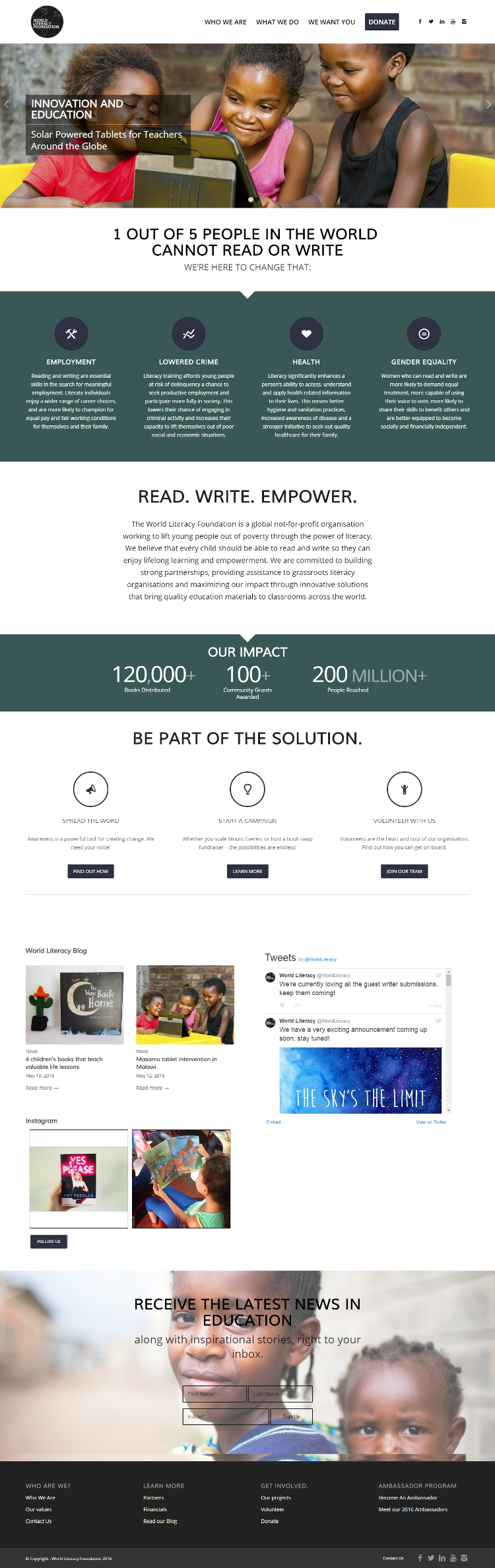The web page for the World Literacy Foundation opens with a striking black circle emblem featuring white letters and a globe design at the top. Navigational tabs for "Who We Are," "What We Do," "We Want You," and "Donate" are prominently displayed. The "Donate" button is highlighted in black with white lettering. There are also social media icons for Facebook, Twitter, and Instagram, along with email and phone icons.

Beneath the navigation bar, a vivid image features three young children: a brown-skinned girl with her hair pulled back in a ponytail, wearing a pink tank top in the center. To her right stands a boy in a black tank top. On the left is a girl with a loose, colored afro, wearing a red scoop-neck T-shirt. Superimposed over this image are the words "Innovation and Education," accompanied by the tagline "Solar Power Tablets for Teachers Around the Globe."

Below the image, a statement reads, "One out of five people in the world cannot read or write. We're here to change it." This is followed by a green banner featuring four icons: a hammer over a wrench labeled "Employment," a graph labeled "Lower the Crime," a heart labeled "Health," and a gender equality symbol. Another section proclaims, "Read, Write, and Empower," framed by another green banner showcasing their impact: "120,000 books distributed, 100+ community grants awarded, and 200 million+ people reached."